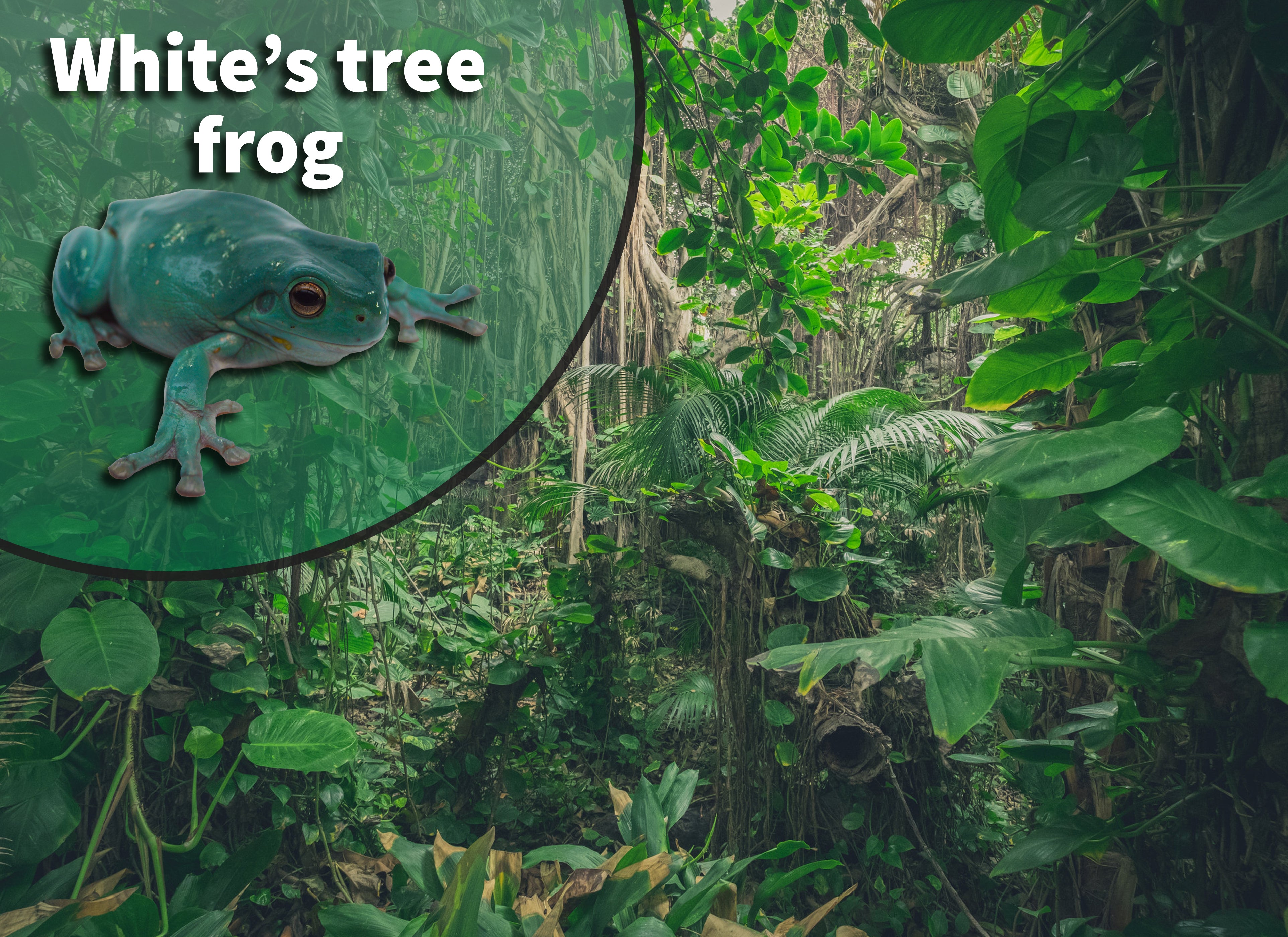The photograph depicts a dense tropical jungle or forest brimming with lush greenery and various plant species. The scene is teeming with life, showcasing abundant ferns, palm-like fronds, and myriad green leafy structures interwoven with vines and branches. In the top left corner of the image, a circular inset highlights a white tree frog. The inset, edged in a transparent green with a black outline, displays the text "White's tree frog" in white font. The frog, which is actually a mint green or dark green color with goldish eyes, appears slightly slimy, reinforcing the moist, verdant habitat that it presumably resides in. The intricate details of the jungle floor are obscured by the dense foliage, further emphasizing the rich, overgrown nature of this vibrant, daytime jungle scene.